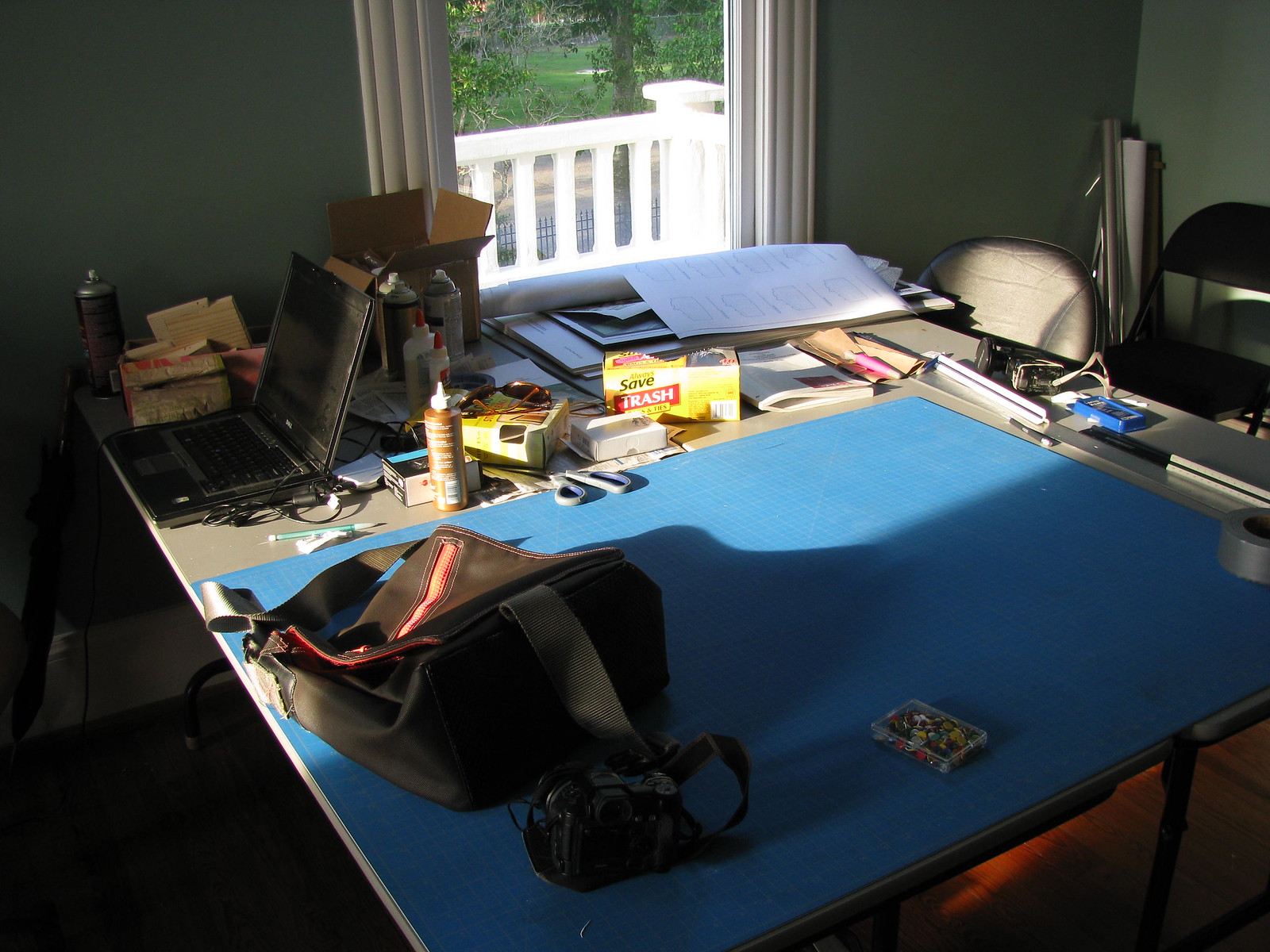A cozy, lived-in home office with an air of creative chaos. The focal point of the room is a large drawing table that resembles an oversized card table, covered in an array of tools and items indicative of a busy, multi-disciplinary project. 

Against the top center wall is an open window with shades drawn up, allowing a view of a white balcony, a black iron gate, and a picturesque landscape of green fields and trees beyond. 

On the drawing table itself, there is a mix of items, including blue graph paper, a camera, a theme board with thumbtacks, a camera bag, a container of trash bags, various rulers, a laptop tangled in wires, a canister, glue, spray paint, and an open box with unseen contents. 

Additional clutter includes what appears to be a makeup bag, a shoebox full of various items, sunglasses, other miscellaneous boxes, a pencil, scissors, manuals, architectural drawings, a roll of blueprints, another unidentified tool, and an open box with its contents spilling onto the cluttered workspace.

Overall, the room is messy, yet it speaks to a dynamic and industrious atmosphere.